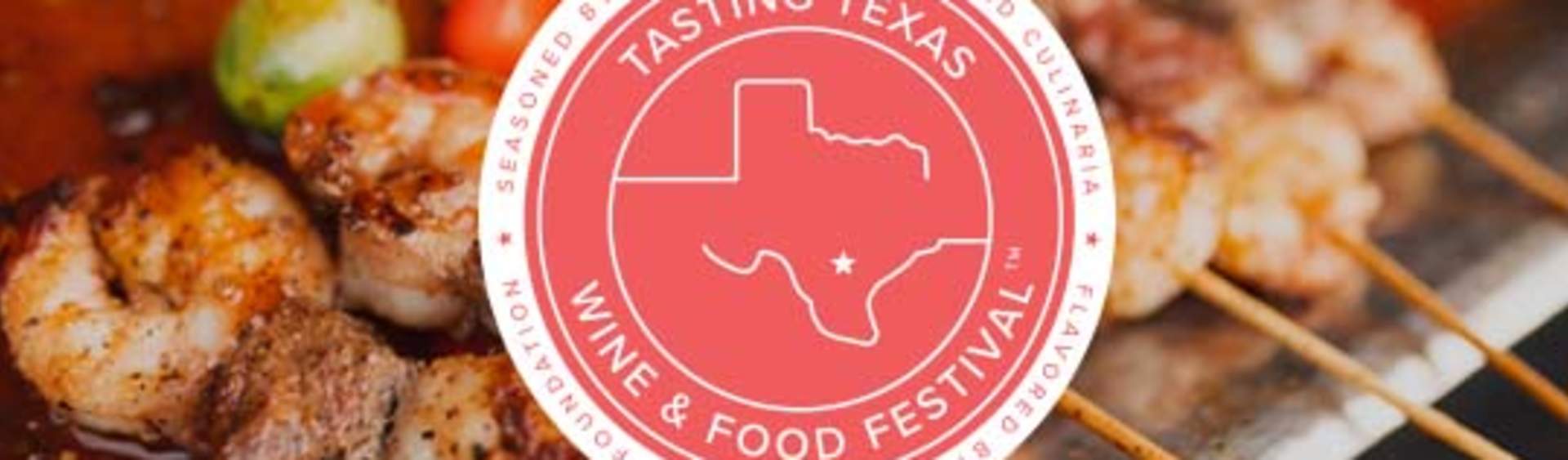This is a detailed photograph focusing on perfectly grilled shrimp kebabs arranged in a row on metallic skewers, possibly extending towards the right. Each kebab skewer is adorned at the top with a green olive and a cherry tomato, showing a delightful golden-brown, well-cooked texture. The image is a long horizontal rectangle with a close-up view, emphasizing the vibrant, appetizing details of the shrimp. The upper left background features a splash of red color, adding to the visual appeal. Central to the image is a circular emblem with a white border and a red center, displaying an outline of the state of Texas with a star towards the bottom. Around the circle, following its border, the text "Tasting Texas Wine and Food Festival" is prominently displayed in white, indicating the theme and event of the photograph.